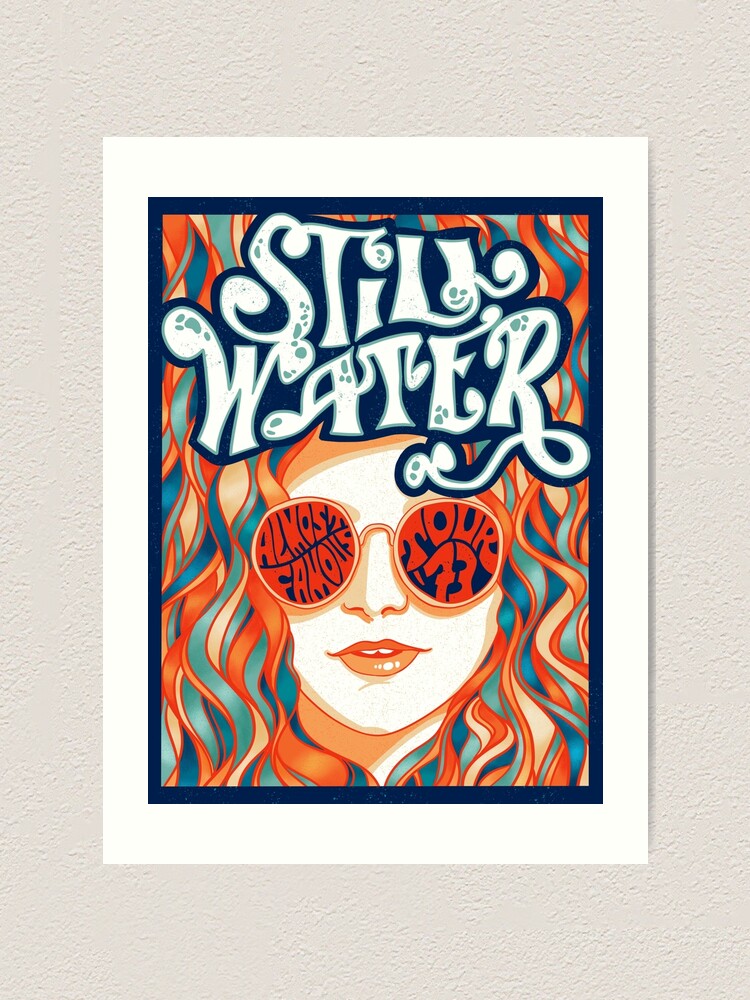The photograph captures a vibrant poster styled in a pop-art theme, prominently featuring a woman with long, curly hair and wearing sunglasses. The sunglasses have red text, with one lens reading "Almost Famous" and the other "Tour 73." Above her head is the name "Stillwater" in large, funky white letters, evoking the late 60s to early 70s rock poster aesthetic. The dominant colors in the artwork are blue, orange, and gold. The artwork is framed with a dark blue border, surrounded by a white frame, and is mounted on a beige, textured stucco wall. The poster advertises the fictional band Stillwater from the film "Almost Famous" directed by Cameron Crowe, with the woman in the image resembling Kate Hudson's character from the movie.